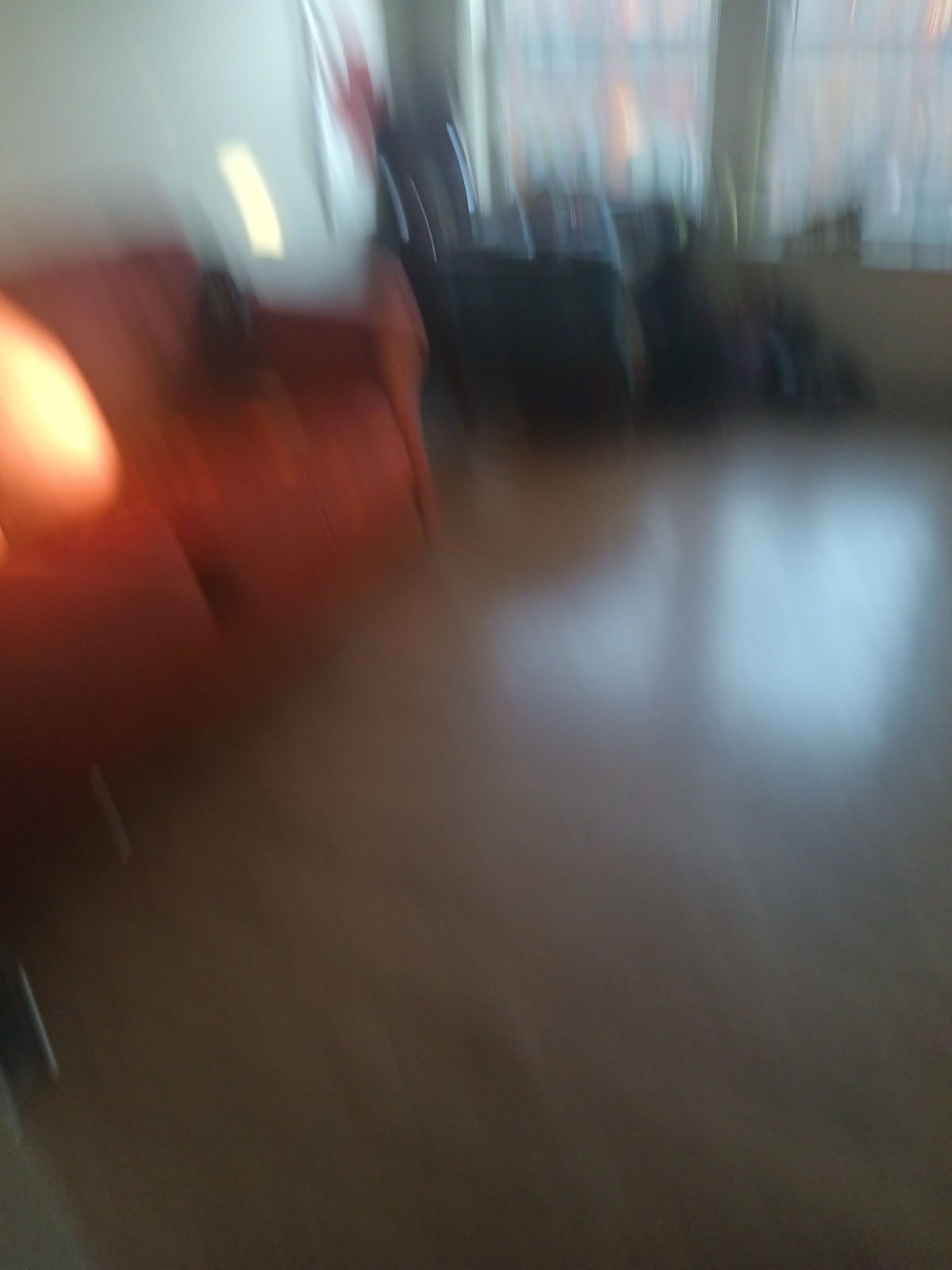A photograph, taken indoors, captures a scene within a living room. The image is extremely blurry and the camera appears to be in motion, making it difficult to discern precise details. However, certain elements can be identified. On the left side of the frame, a red couch or loveseat is positioned against a wall. A bright spot of sunlight or possibly the glow from a lamp illuminates the back cushion of the couch. To the right, against another wall, are two windows through which another building is faintly visible. In front of the windows, there is an indiscernible, large, dark shape that might be a piece of furniture or multiple items, colored in very dark brown or black. The floor appears shiny, reflecting light coming from the windows, adding a reflective quality to the scene. Despite the blurriness, the overall atmosphere of an empty and quiet living room is conveyed.